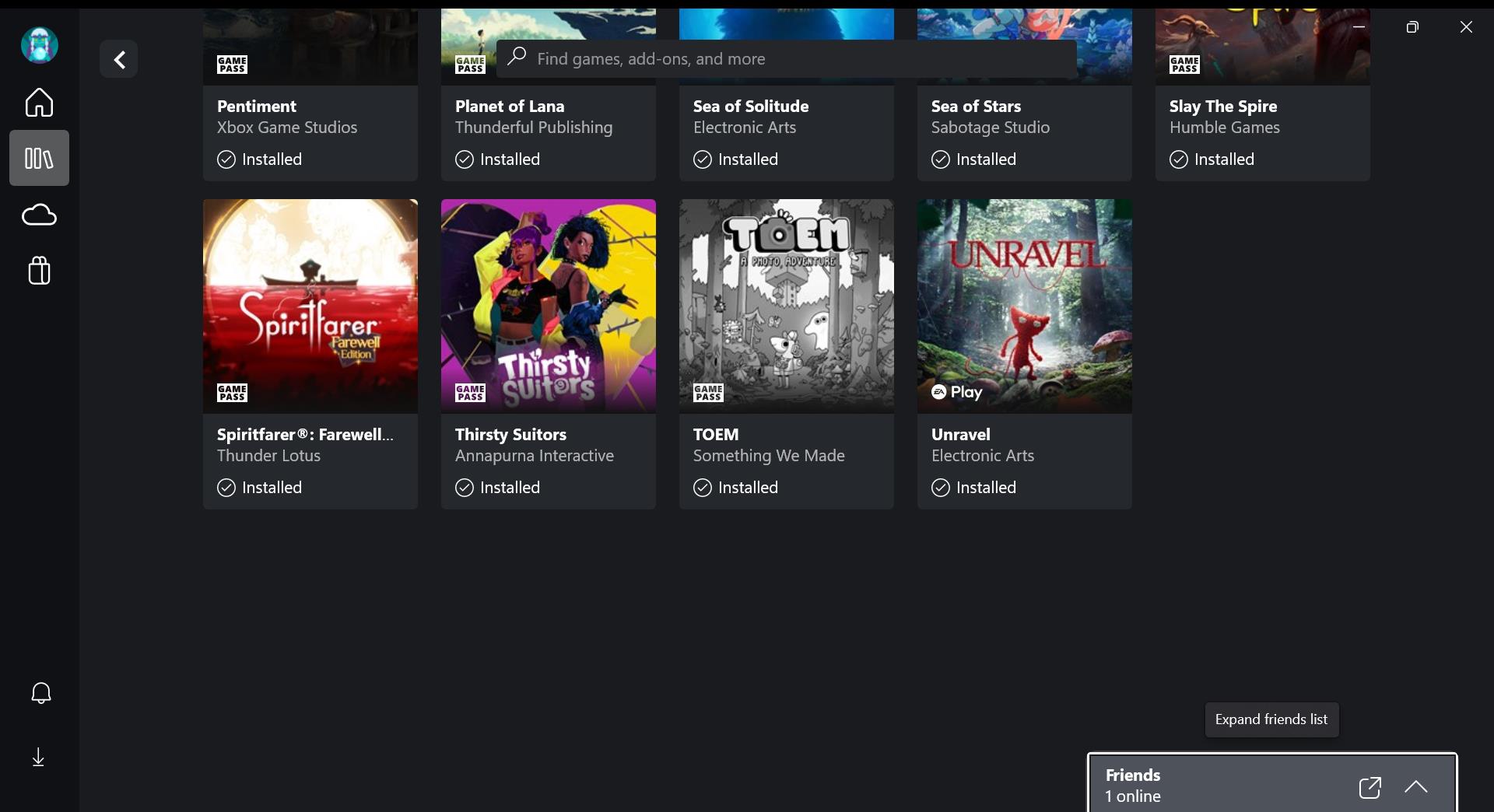The image features a black background as its main canvas. On the left side, there is a small blue circle displaying a person's face, followed by an icon of a house immediately next to it. Below these, there are icons that resemble stacks of books or movie reels, a cloud icon, and a bag icon. Moving to the bottom of the image, there is a bell icon and a thin horizontal line. In the upper right section, there is a left-facing arrow, and a text label that reads "Find games, add-ons, and more." Just beneath this text, the lower parts of several game icons are visible, including titles such as "Spiritfarer," "Thirsty Suitors," and "Unravel."

At the bottom of the image, there is a gray button labeled "Expand search list," along with another gray button that reads "Friends (1 online)." Beside this second button, there is a small white box featuring an upward-pointing arrow.